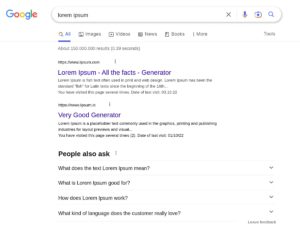The image depicts a blurry screenshot from Coakley's search engine, showing search results for the term "Lauren Ipsum" entered in the search bar. There are two primary web results visible. The first result titled "Lauren Ipsum on the Fact Generator" is presented in blue text, indicating it is a clickable link. However, the description and URL for this result are blurry and unreadable.

The second result is titled "Very Good Generator" and is highlighted in purple, suggesting it has been clicked before. Similar to the first, its description and URL are also blurred and difficult to decipher.

At the bottom of the image, there is a section labeled "People also ask" featuring four common questions. Out of these, only the second question, "What is Lauren Ipsum good for?" is readable, though the rest of its text remains unclear. The remaining three questions, including "How does Lauren Ipsum work?" and "What does the word Lauren Ipsum mean?" are partially visible but mostly obscured.